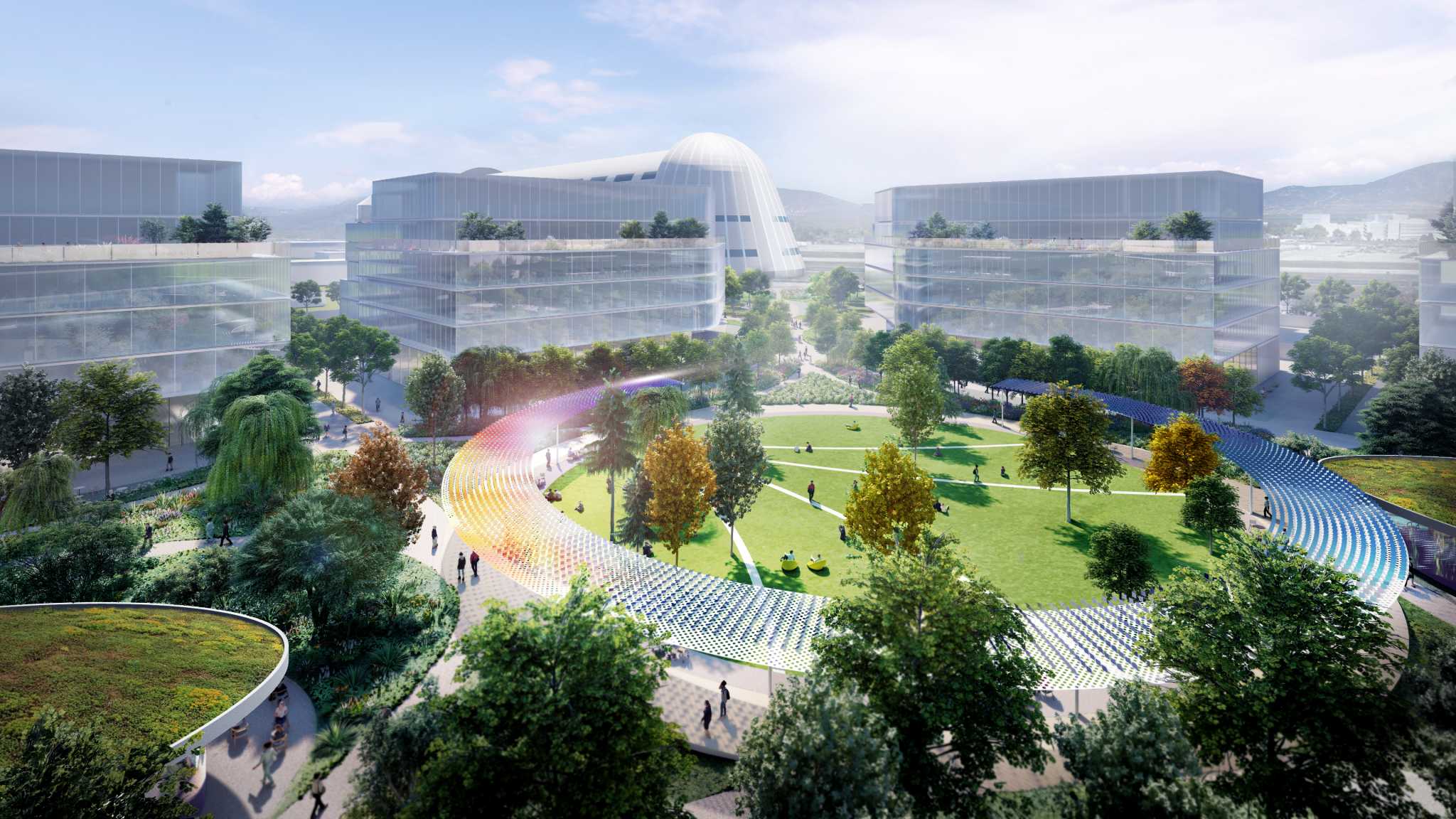The image is a computer-generated, futuristic mock-up of an outdoor community, viewed from a slightly elevated, bird's-eye perspective. It features three distinct, transparent buildings with glass roofs that gleam under a bright, sunny sky with blue hues and scattered white clouds. Each building has grassy areas on its rooftops, with the surrounding grounds abundantly lined with trees in various arrangements.

A central circular courtyard is meticulously landscaped, featuring a grassy field intersected by four pathways and scattered with eight trees. Encircling this courtyard is a silver-trimmed pathway. In the background, a dome-shaped structure extends like a train, adding to the scene’s modernistic ambiance. The vibrant community has people casually walking along the pathways, enjoying the well-designed, tree-filled environment. The overall impression is one of a bright, sunny day in a thriving, green, and futuristic neighborhood.